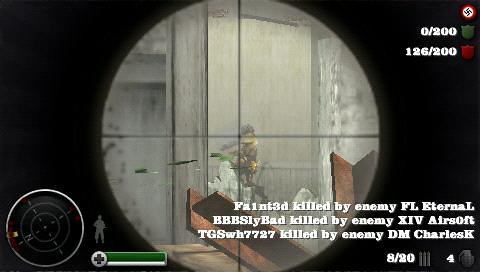The screenshot captures an intense, action-packed moment from a World War II-themed video game. At the center of the image, the player is gazing through the crosshairs of a sniper rifle. The sniper scope features pencil-thin, intersecting vertical and horizontal black lines, creating a circular view while the surrounding area remains blacked out, except for game elements overlaying the screen. The crosshairs are precisely aimed just to the left of the head of a distant character dressed in military-style camouflage, seemingly walking to the left near a doorway or window framed by gray walls.

The top right corner displays a prominent black swastika inside a white circle on a red background, reinforcing the WWII setting. Nearby, a green shield icon reads "0/200," and a red shield icon shows "126/200." In the bottom right corner, a series of white text reveals player updates such as "Faint3D killed by enemy FLEternal," "BBBSLIbad killed by enemy XIVAirsoft," "TGSwish7727 killed by enemy DMCharlesK," followed by "8/20" and the number "4." Additionally, the lower left of the image features a map icon, and to its right, a rectangular green health bar marked with a plus sign, which appears to be fully charged.